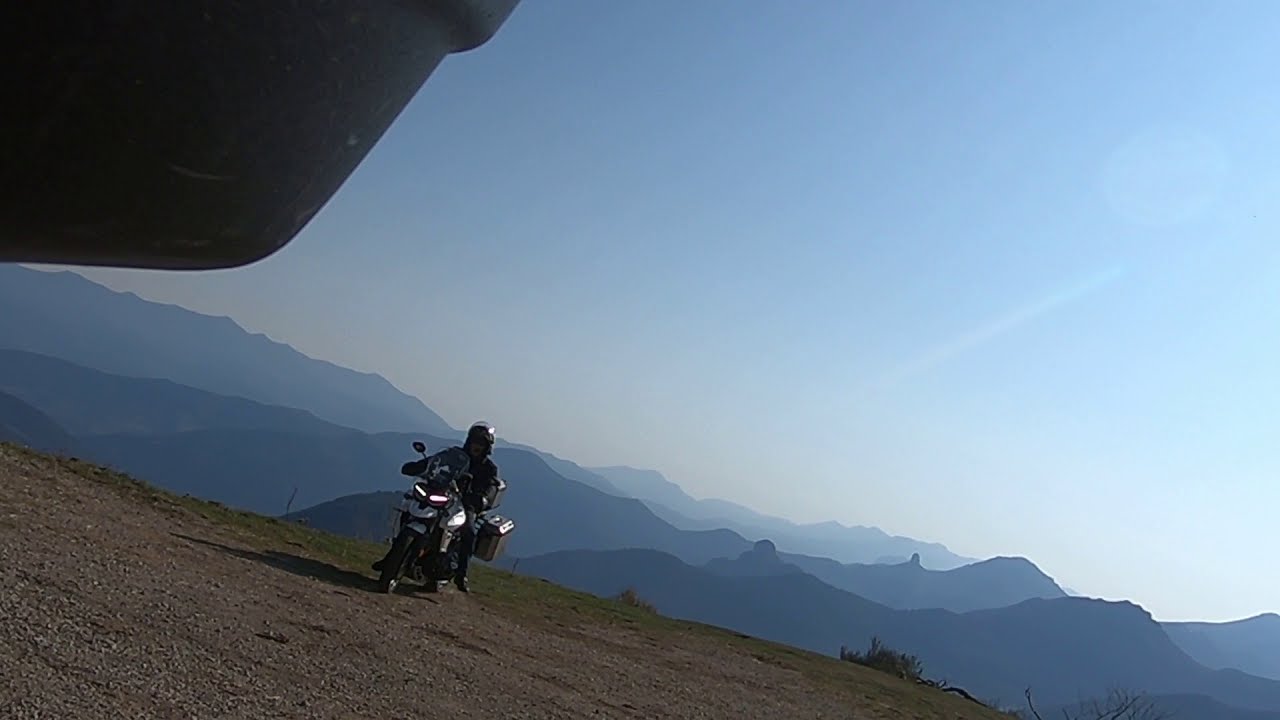In this wide, rectangular photograph, a rider on a touring motorcycle is positioned in the bottom left quadrant, slightly facing the camera. The rider, attired in full motorcycle regalia including a helmet, leather jacket, and long pants, sits on a grayish brown dirt patch with small gray rocks that gradually become grassier towards the horizon. A mountainous landscape serves as the backdrop, with a range of silhouetted peaks fading from darker blue in the foreground to lighter blue in the distant background. The horizon line begins midway on the left side of the photograph and angles downward to the bottom right corner, adding a dynamic diagonal element to the composition. Above this scene, a clear, light blue sky stretches across the upper portion of the image. In the top left corner, a black metallic object, likely part of another motorcycle's baggage compartment, partially obstructs the view. Overall, the picture captures a serene moment of a motorcyclist pausing amidst vast, impressive mountain landscapes.